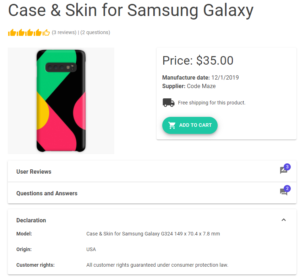**Detailed Product Listing Description:**

This product listing is displayed within a square image frame set against a clean white background. Dominating the top section of the listing is large, bold text that reads "Case and Skin for Samsung Galaxy," integrating a header that stands out prominently. Just below this header, the listing boasts a four-star rating indicated by four thumbs-up icons. Although the specific view count and question numbers are present, they are not legible due to the small size of the text.

Central to the listing is an illustrative image of the Samsung Galaxy phone case, which features a striking design with a black background adorned with vibrant green and pink splashes. This eye-catching color combination adds a pop of brightness and modern flair to the product.

To the right of the product image, a price box is prominently displayed, marking the cost of the phone case at $35. Within the same area, additional details such as the manufacturer date and supplier are mentioned, though specifics are not provided. Enhancing the usability of the listing, a green "Add to Cart" button is strategically placed for easy access.

Beneath this main section, a series of horizontal lines organizes supplementary information. This section includes tabs for user reviews, questions, and answers, allowing potential buyers to engage with feedback and inquiries about the product. Additionally, further down, there are declarations regarding the model, origin, and consumer rights, providing a comprehensive overview to ensure customer transparency and satisfaction.